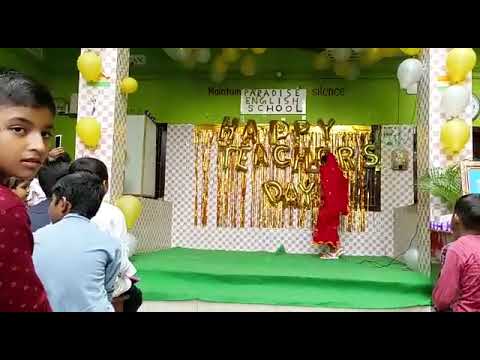The photograph depicts a vibrant celebration at Paradise English School, captured in a landscape orientation with a black border above and below the image. At the center of the stage, which is covered in green carpeting, stands a teacher adorned in a traditional red Hindi sari and veil costume. Behind her, gold balloons spell out "Happy Teacher's Day," complemented by gold streamers, with a smaller sign overhead indicating "Paradise English School." The stage is further embellished with yellow and white balloons on either side and hanging from the ceiling. The backdrop includes a white wall with gold fringes and a larger green wall beyond. In the foreground, several Indian children are seated, attentively facing the teacher, except for one young girl in a red shirt on the left, who has turned towards the camera. The scene likely captures the teacher in the midst of a presentation, with the festive decorations and attentive audience underscoring the significance of the occasion.